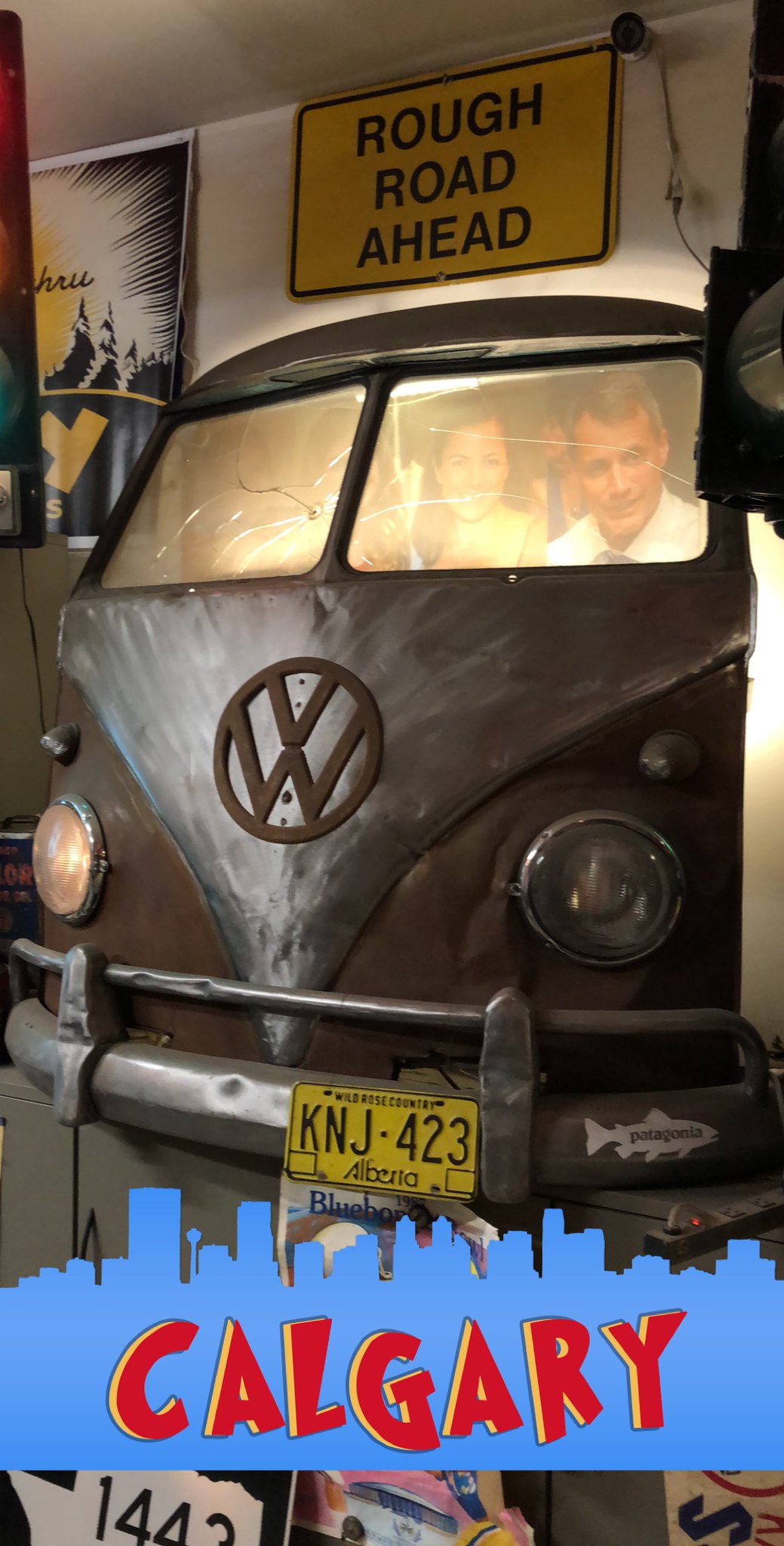In this captivating museum exhibit, a striking display features an old Volkswagen Vanagon bus prominently positioned against a white wall background. The interior of the bus is lit up, revealing hanging pictures of a man and a woman. Its left headlight shines brightly, creating a guiding light effect, while the right one remains unlit. The front of the bus proudly showcases a yellow Alberta license plate that reads "Wild Bros Country KNJ 423" and a Patagonia bumper sticker. 

Above the bus, a distinctive yellow sign declares "Rough Road Ahead," seemingly hanging out of the wall, indicating a journey to come. On the left side, a partially visible poster hints at additional artwork, adding to the curiosity of viewers. Beneath the Vanagon, there's a blue silhouette of a city skyline with bold red and yellow text that proclaims "Calgary." The colors in the scene include a mix of white, red, black, yellow, gray, brown, and light blue, all combining to create an intriguing and detailed visual narrative.